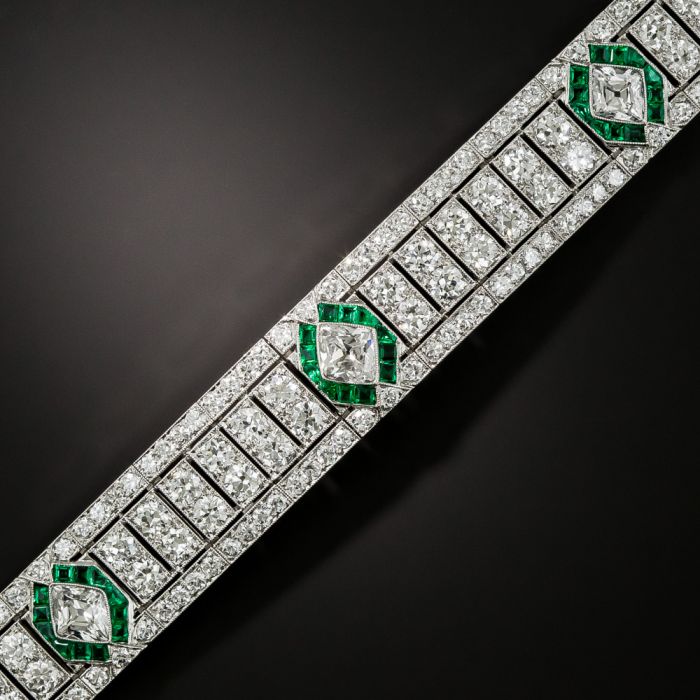The image captures a close-up of an exquisitely detailed jewelry belt or bracelet, elegantly draped across a dark gray background, spanning from the bottom left to the top right corner of the frame. This luxurious piece features numerous small diamonds arranged in two parallel channels along the outer edges. Positioned between these channels are six rows of pairs of larger diamonds. Amidst these rows, a pattern emerges: in the middle section, three prominently larger diamonds, each nestled within a cluster of green emeralds, punctuate the design at regular intervals. The craftsmanship is pristine, showcasing a dynamic and rich appearance that makes the jewelry piece stand out with an aura of sophistication and opulence. The image displays this intricate pattern thrice, enhancing the allure and elegance of this timeless piece, which epitomizes refined luxury and meticulous design.